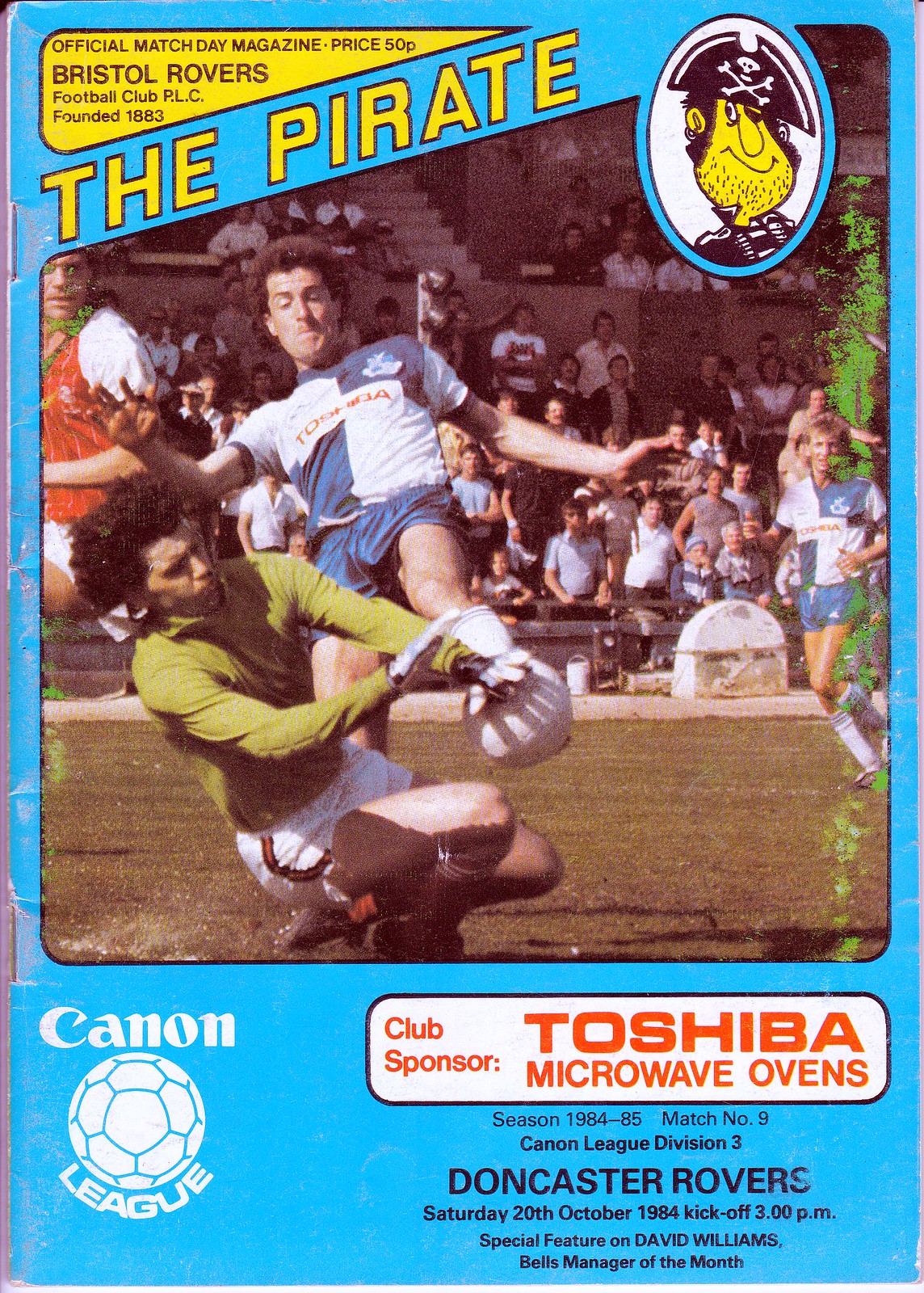The cover of this official match day magazine for the Bristol Rovers Football Club, founded in 1883, is a vivid and detailed layout. The primary background color is light blue, and you can see staples on the left side, indicating the magazine's binding. The very top left corner features a yellow triangular banner with black text reading, "Official Match Day Magazine, Price 50p, Bristol Rovers Football Club, PLC, founded 1883." 

Just below this, in bold yellow text with a black border, is the title "The Pirate" on a blue background. To the right of the title, a white oval contains a detailed cartoon graphic of a pirate. The pirate dons a black hat featuring a white skull and crossbones, has yellow skin, black hair, a 5 o'clock shadow, and is wearing a black jacket.

Beneath the cartoon, a photograph captures the intensity of a soccer game in progress. At the center left, a player in a white and blue jersey kicks the soccer ball, while a goalkeeper in an olive green jersey dives low, extending a hand to block the kick. The scene is set on a dark green soccer pitch, surrounded by spectators in the stands. Additional players can be seen at the very left and the very right of the image.

At the bottom of the cover, on a blue background, the Canon logo alongside a white soccer ball labeled "League" appears on the left. To the right, a white rectangle with red text reads, "Club Sponsor Toshiba Microwave Ovens." Below, in black text on a blue background, further details are provided: "Season 1984-85 Match No. 9, Canon League Division III, Doncaster Rovers, Saturday, 20 October 1984, kickoff 3 p.m. Special feature on David Williams, Bell's Manager of the Month." The photograph appears somewhat scuffed, likely from age, with a greenish discoloration at the very right, not part of the original image.